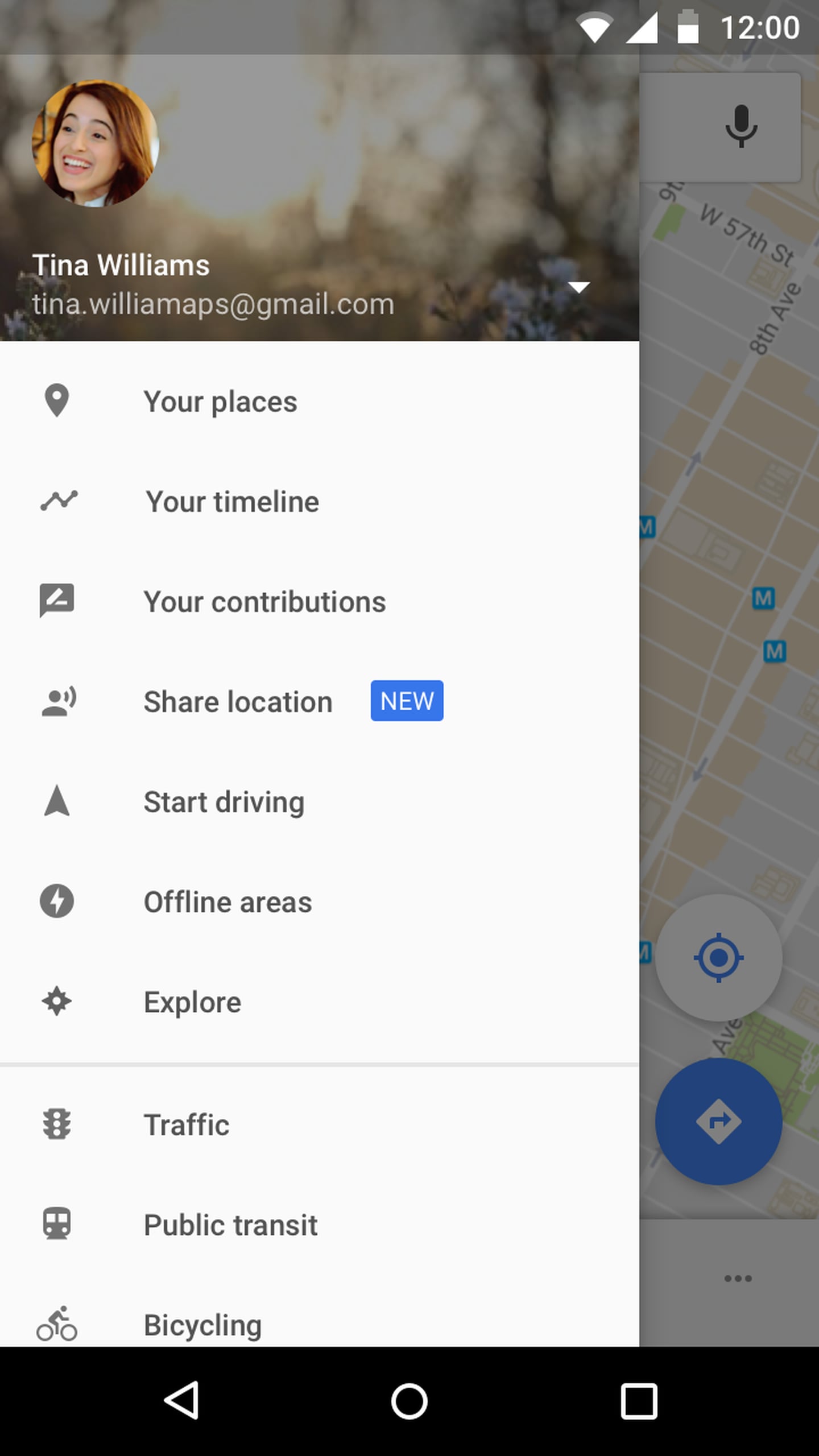The screenshot displays a mobile website interface. The background, which appears to be a map, is obscured by a central pop-up window that takes precedence over the rest of the screen. 

At the very top of the screen, the device's status bar is visible, showing the current time (12:00), Wi-Fi signal strength, cellular signal strength, and battery level.

The pop-up window has a white background and a roughly rectangular shape. Inside the pop-up, a user's profile information is prominently displayed. The profile section starts with a circular image of the user's face, followed by the user's name, "Tina Williams," with proper capitalization. Below the name, her email address is partially visible, formatted as "tina.williams@gmail.com," albeit with "WILLIAMAPS" instead of the correct email suffix.

Beneath the profile details, there is a down arrow symbol, suggesting a dropdown or expandable menu. The left side of the pop-up is lined with several icons that are vertically stacked.

The main body of the pop-up lists various options, delineated by category headers and separated by lines. The options presented include:

1. **Your Places**
2. **Your Timeline**
3. **Your Contributions**
4. **Share Location** (Highlighted with a small blue label reading "New")
5. **Start Driving**
6. **Offline Areas**
7. **Explore**

A horizontal divider is then followed by additional options:

1. **Traffic**
2. **Public Assist**
3. **Isolating**

The design is clean, allowing easy navigation through the various options and features available to the user on this mobile interface.